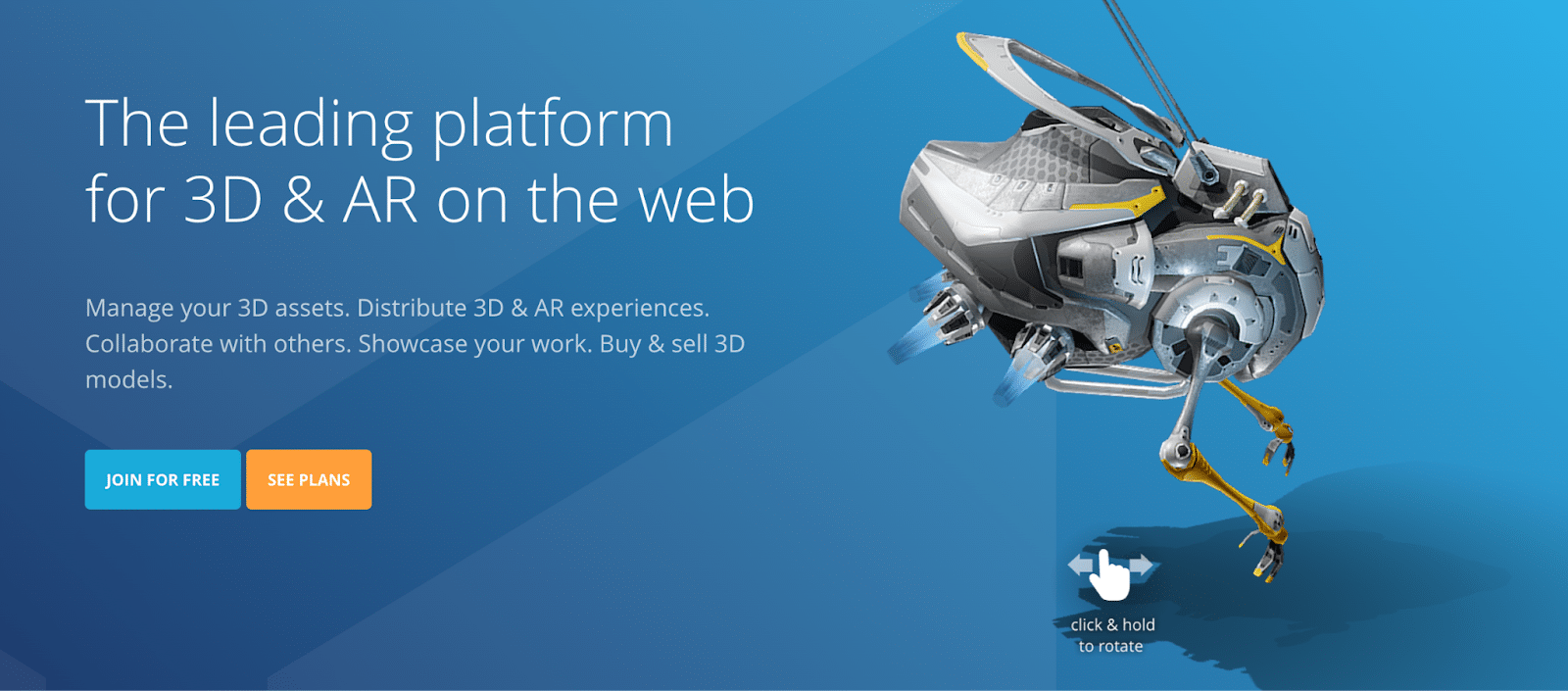The image features a vibrant blue background with crisp white text prominently stating its purpose: "The Leading Platform for 3D and AR on the Web." The text elaborates on the platform's capabilities, including the ability to manage 3D assets, distribute 3D and AR experiences, collaborate with others, showcase work, and buy and sell 3D models. Below this informative content are two buttons: a blue one labeled "Join for Free" and an orange one labeled "See Plans."

Adding a whimsical element to the scene is a silver electronic character with an open lid, accented by little yellow trims and bent yellow legs. The character also features touches of blue along the edges, giving it a futuristic feel. Adjacent to this character is a hand with one finger pointed up, accompanied by arrows pointing in both directions and an instruction that reads, "Click and hold to rotate," inviting users to interact with and explore the character's features from all angles.